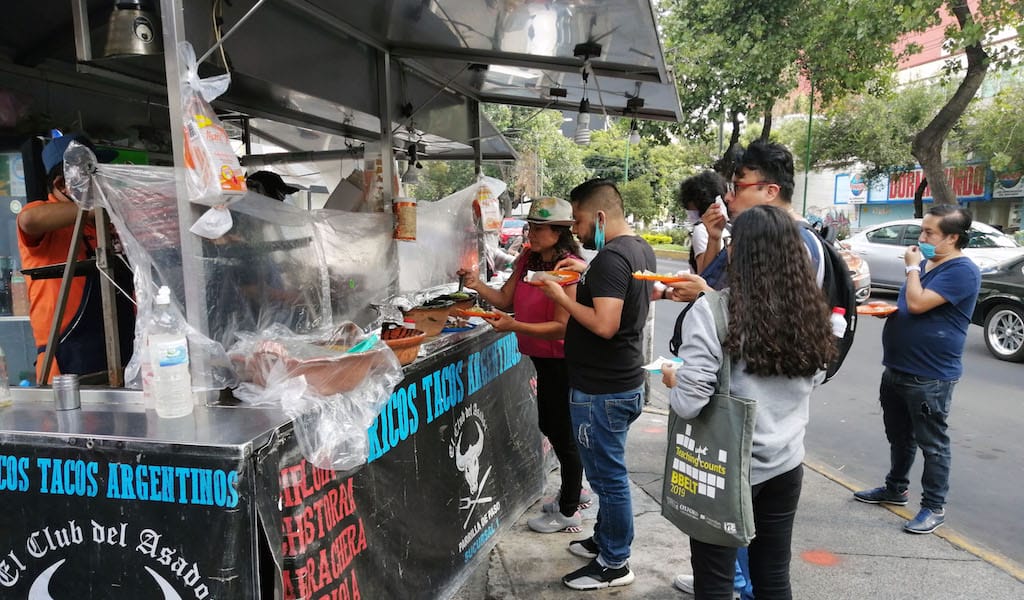The photograph captures a vibrant street food scene in an urban setting, likely a suburban city, given the presence of trees and cars in the background. At the heart of the image is a bustling food cart with a steel roof, distinctly labeled as "Marcos Tacos Argentinas," suggesting it serves Argentinian cuisine. Multiple baskets of food are displayed on the front of the cart. Six customers are visible, enjoying their meals on orange plates.

In front of the food cart, a woman in a pink shirt with a beige hat stands out, accompanied by a man with dark hair, a beard, and a black t-shirt, whose mask dangles from his ear as he eats. Beside them is a casually-dressed girl with wavy hair, sporting a grey bag with a white and yellow design, alongside a taller man with red glasses. A bit further back stands a blue-shirted man with black jeans, a protruding tummy, and a blue mask.

Inside the cart, two workers are visible, attired in orange shirts, blue aprons, and blue hats. A large plastic sheet separates the workers from the customers, likely a precaution for infection control measures. This clear barrier does not impede the lively interaction between the food cart staff and the hungry patrons, enhancing the bustling, yet organized atmosphere of this urban street food haven.